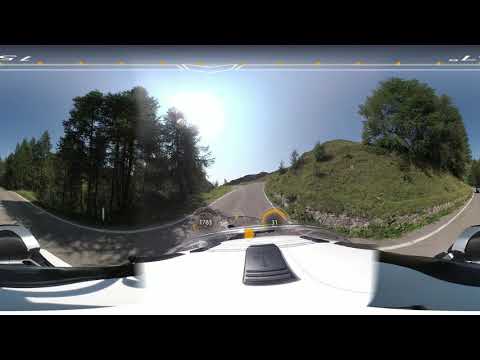The image shows a distorted, panoramic view captured using a fisheye lens, taken from the perspective of a white RV, likely with a GoPro or similar camera mounted on its hood. The central road, made of gray asphalt, stretches ahead and curves both left and right, creating a unique, warped appearance. On the right side of the road, there is a grassy hill underpinned by a foundation of rocks. The landscape is complemented by various green elements, including pine trees, bushes, and wild grass. Above, a bright sun dominates the clear, blue sky with no visible clouds, suggesting a sunny, cloudless day. The overall scene conveys a sense of traveling through a rural or suburban area, with natural, unmanicured surroundings.